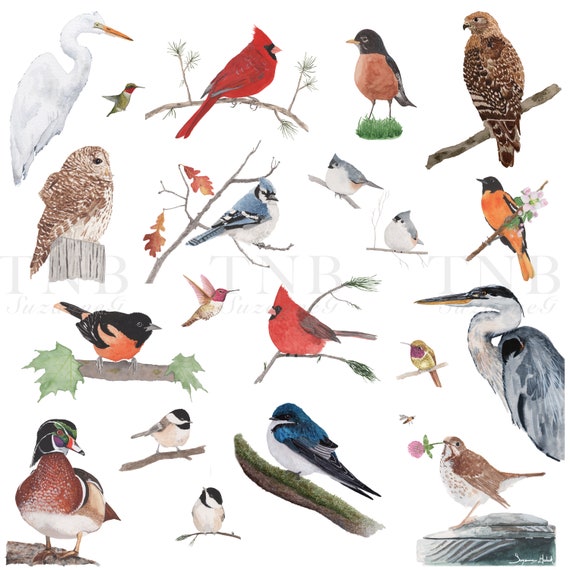This image, resembling a page from a birding book, features a collection of watercolor-styled bird illustrations arranged in rows, set against a white background with a faint watermark and partial script reading "TNB." In the top left corner, there is a large white Great Egret with a yellow beak facing right, next to a small hummingbird. Below these, a brown owl perches on a stump, and an orange and black Baltimore Oriole is visible on a tree branch underneath. A brown and white duck is depicted below, followed by a series of birds to the right: a male Northern Cardinal with a mohawk-like crest sitting on a stick, and below it, a Blue Jay also perched on a stick. Further along this row are another hummingbird and two chickadee-like finch birds. In the bottom-right section, a blue and white bird stands on a piece of grass, accompanied by another Northern Cardinal, two more finch-like birds, a brown and black bird, and a brown hawk on a branch. A yellow and black bird perches nearby, and another egret, this time gray, is depicted along with a small brown and white thrush holding a pink flower in its beak.